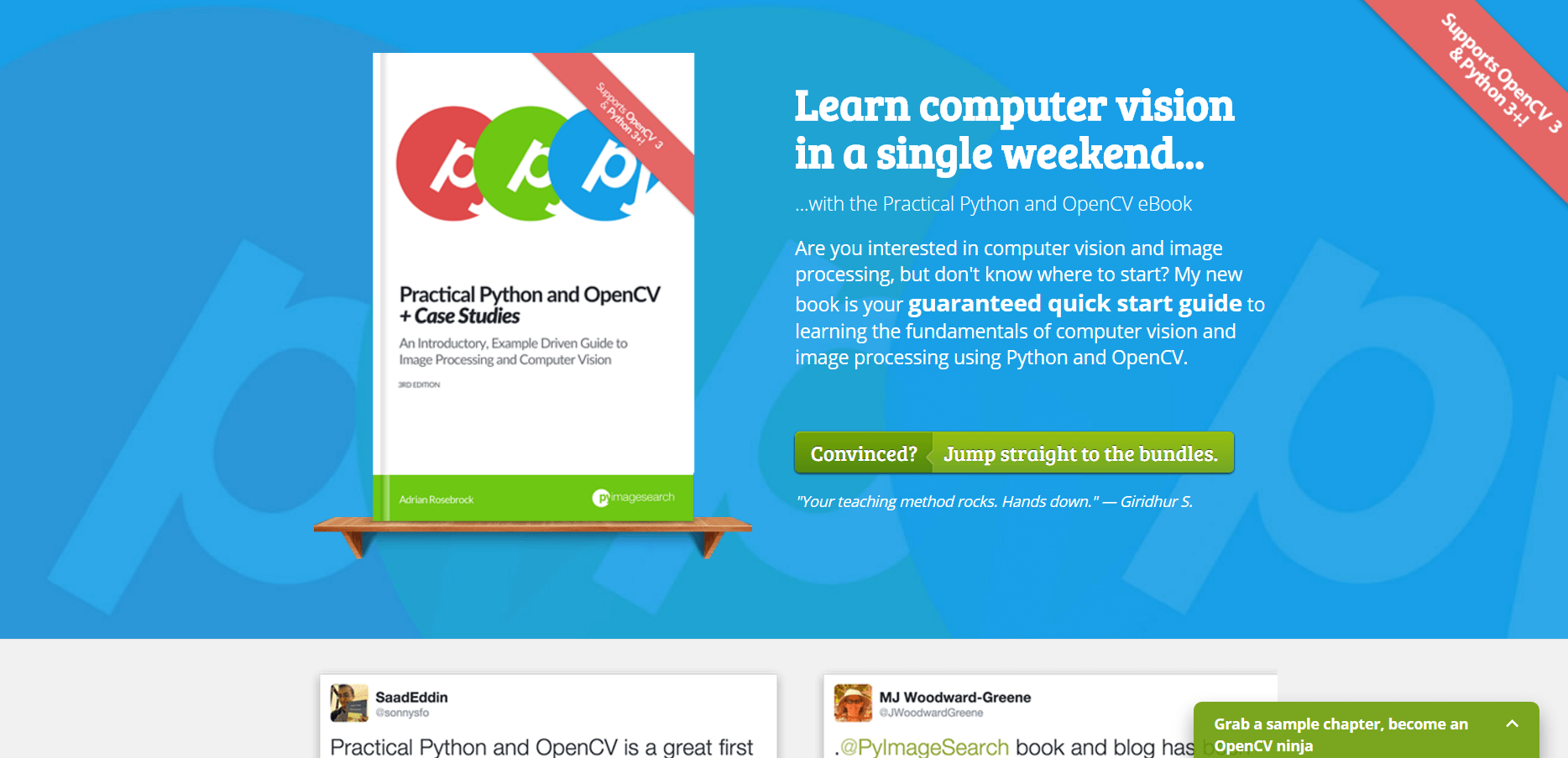**Ad for Computer Class:**

The advertisement boasts a clean and visually appealing light blue background. Subtly integrated into this backdrop are letters in a slightly different shade of blue forming 'P, P, and P.' In the foreground, the main focus is a white book resting on a wooden shelf. The book features a contrasting green banner at the bottom with the name "Adrian Rosebrock" and "PyImageSearch" inscribed on it. An orange diagonal banner at the top of the book catches attention, displaying the text "Supports OpenCV 3 and Python 3+!"

Prominently displayed on the book cover are three overlapping circles colored red, green, and blue, each containing a white 'P' and a partial 'Y' visible in the last circle. Below these circles is the book's detailed title: "Practical Python and OpenCV in Case Studies: An Introductory Example-Driven Guide to Image Processing and Computer Vision, 3rd Edition."

Adjacent to the book, a bold white text reads: "Learn Computer Vision in a Single Weekend." Below this is an ellipsis followed by the phrase "with the Practical Python and OpenCV ebook." A call to action entices potential readers: "Are you interested in computer vision and image processing but don’t know where to start? My new book is a guaranteed quick start guide to learning the fundamentals of computer vision and image processing using Python and OpenCV."

Further engagement is encouraged with a green banner stating "Convinced" in white, set against an olive background. Beside it, another banner with a light green background reads: "Jump straight to the bundles" in white font. A testimonial statement below praises the teaching method: "Your teaching method rocks. Hands down." — @erdars.

In the upper right corner, another orange banner reiterates: "Supports OpenCV 3 and Python 3+!" in white text. Underneath, snippets from social media posts feature the authors' names and partial reviews, adding an additional layer of credibility to the book and the course being advertised.